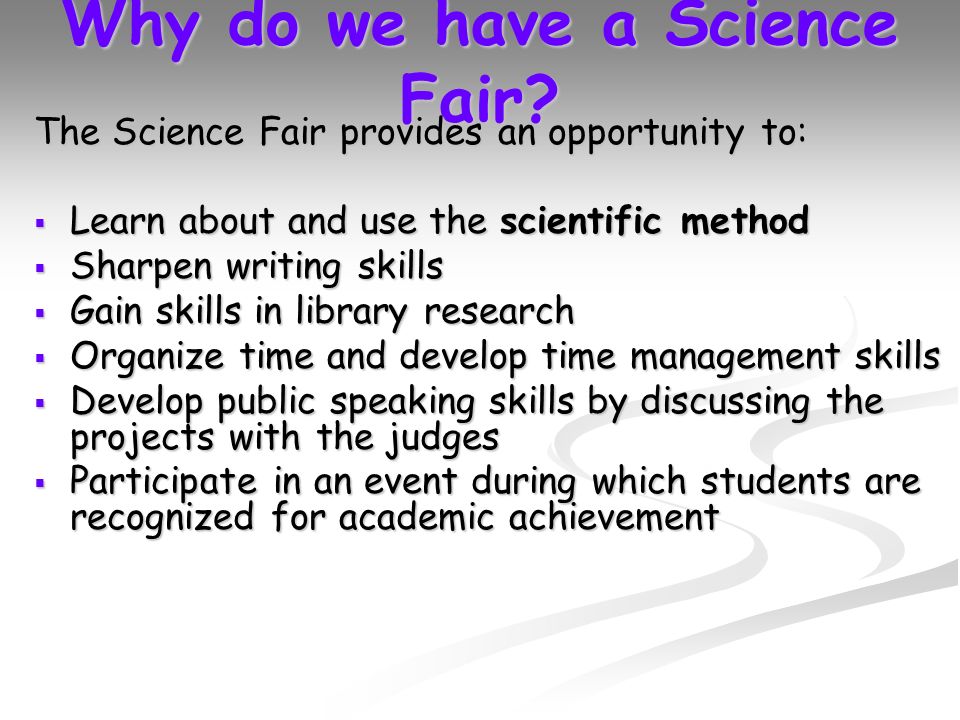This image resembles a PowerPoint slide with its rectangular shape and width longer than its height. The background starts as a dark gray at the top, gradually transitioning into lighter gray and finally white at the bottom. In the lower right corner, gray wave patterns form shapes resembling 'SS' with a 3D effect. Dominating the slide is the title in large purple text with a subtle white shadow, "Why do we have a science fair?". Below the title, in smaller black font, the text reads: "The science fair provides an opportunity to..." followed by several bullet points also in black text. These points include: learning about and using the scientific method, sharpening writing skills, gaining skills in library research, organizing time and improving time management skills, developing public speaking skills by discussing projects with judges, and participating in an event where students are recognized for academic achievement. Adjacent to these bullet points on the left are small purple squares with gray shadows, matching the color of the title text.